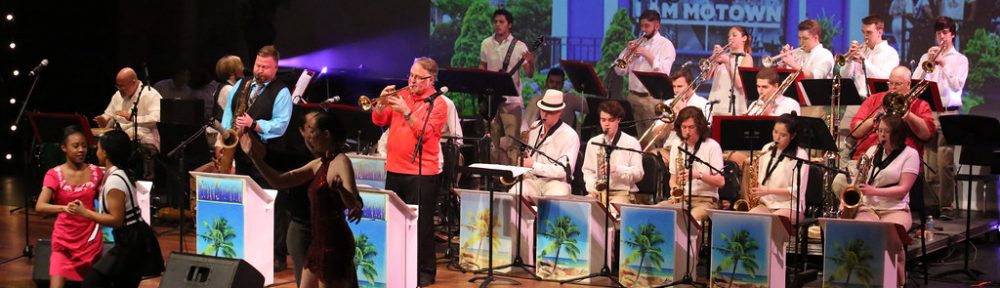The photograph captures a vibrant scene of a jazz band performing on a stage. The backdrop prominently features the words "Moe Town" in white. In the front row, a man with glasses and wearing orange appears to be the focal point, possibly playing the clarinet. He is flanked by another musician in blue with a vest and a third individual in white, looking down at something.

Behind them, arranged in several rows, are the other band members. To the right, seated individuals play various instruments including five trumpeters in the back row, followed by a row of trombone players with their distinct long slides. The front row is composed of woodwind players, including clarinets, oboes, and saxophones.

In front of the instrumentalists, a black desk holds their sheet music. The band is marked by a pattern of blue designs on their podiums. Adding to the lively atmosphere, a couple is seen dancing in the background. The couple, two women, one in a pink dress and another in a white dress holding a purse, are holding hands. On the left side of the image, two people are seen socializing, possibly not part of the band.